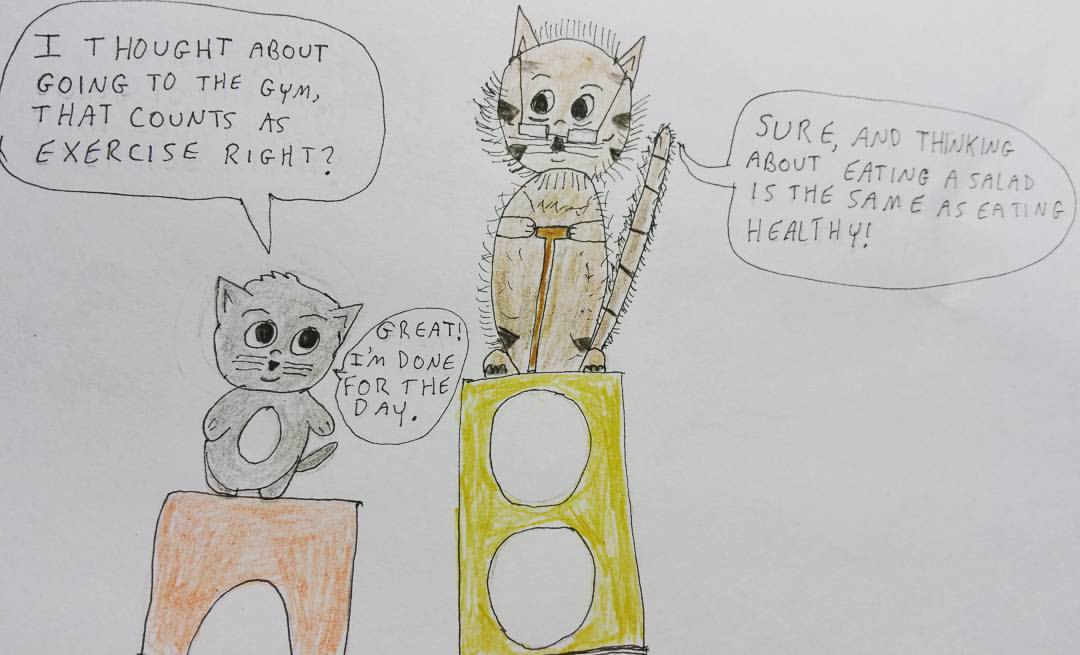This is a hand-drawn cartoon on a white piece of paper, created using markers and ink. On the left side, a gray cat with a white belly stands on an orange cat tree, its round head and belly giving it a cute appearance. It has an open mouth, suggesting it’s talking. This cat has two speech bubbles around it; the first one, placed just above, reads, "I thought about going to the gym. That counts as exercise, right?" The second, positioned to its right, states, "Great, I'm done for the day."

On the right side of the image, a beige cat with a very long tail, adorned with tiger stripes, stands on a higher yellow cat tree with two white cutouts. This cat, drawn with glasses and possibly holding a brown cane, also has its mouth open. It has a speech bubble to its right that says, "Sure, and thinking about eating a salad is the same as eating healthy."

The cartoon humorously depicts the two cats discussing dieting and exercise, with a blank white background emphasizing the characters and their conversation.